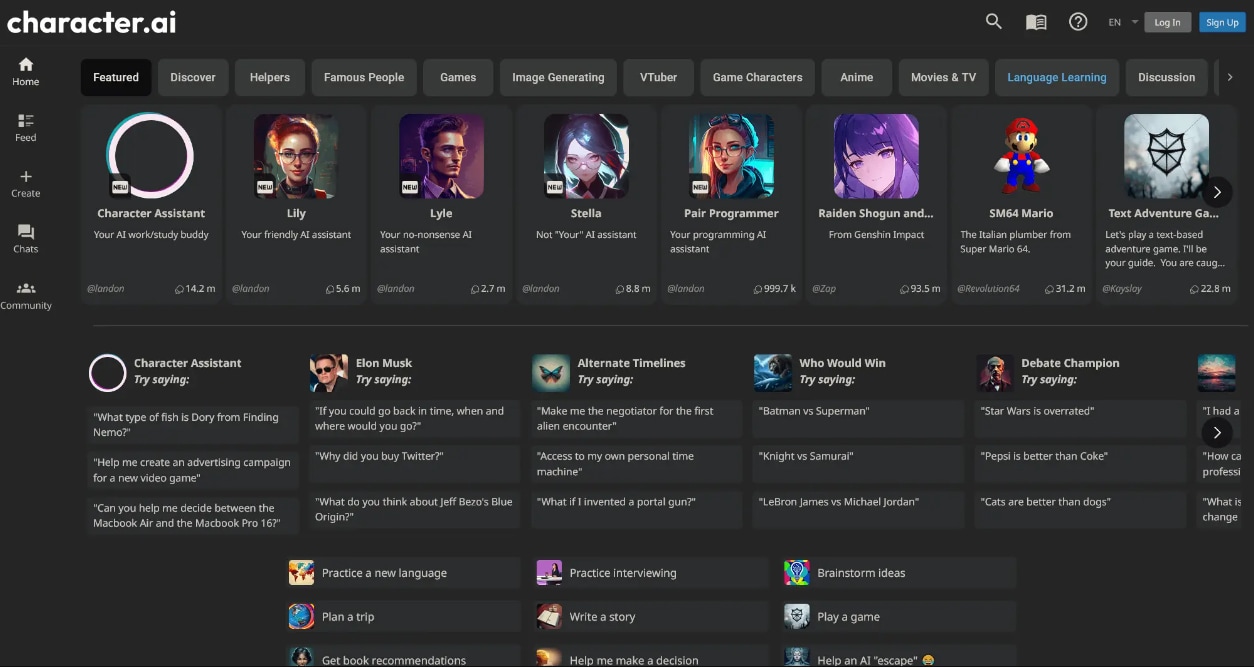The image is a detailed screenshot of a computer screen displaying the Character.ai website. The background of the website is black, providing a striking contrast to the light gray text. In the upper left corner, the site’s name, "Character.ai," is prominently displayed in white. The top-right corner features buttons for "Login" and "Sign Up."

At the very top of the page, a series of navigation tabs are visible, offering a variety of sections: Featured, Discover, Helpers, Famous People, Games, Image Generating, VTuber, Game Characters, Anime, Movies and TV, Language Learning, and Discussions. The "Featured" section is currently selected, indicated by a distinct highlight, while the "Language Learning" tab is marked in blue, suggesting it might be a new or popular section.

Beneath these tabs, there is a horizontal row of images representing different characters or categories. These include "Character Assistant," "Lily," "Lyle," "Stella," "Hair Programmer," "Raiden Shogun," "SM64 Mario," and a "Text Adventure."

On the left side of the screen, there are navigational icons indicating options for "Home," "Feed," "Chats," and "Participants." At the bottom of the screen, various sections provide topics and suggestions, featuring discussions about "Elon Musk," "Alternate Timelines," and hypothetical matchups like "Who Would Win." Additionally, the "Character Assistant" appears to offer personalized suggestions to the user, enhancing the interactive experience of the site.